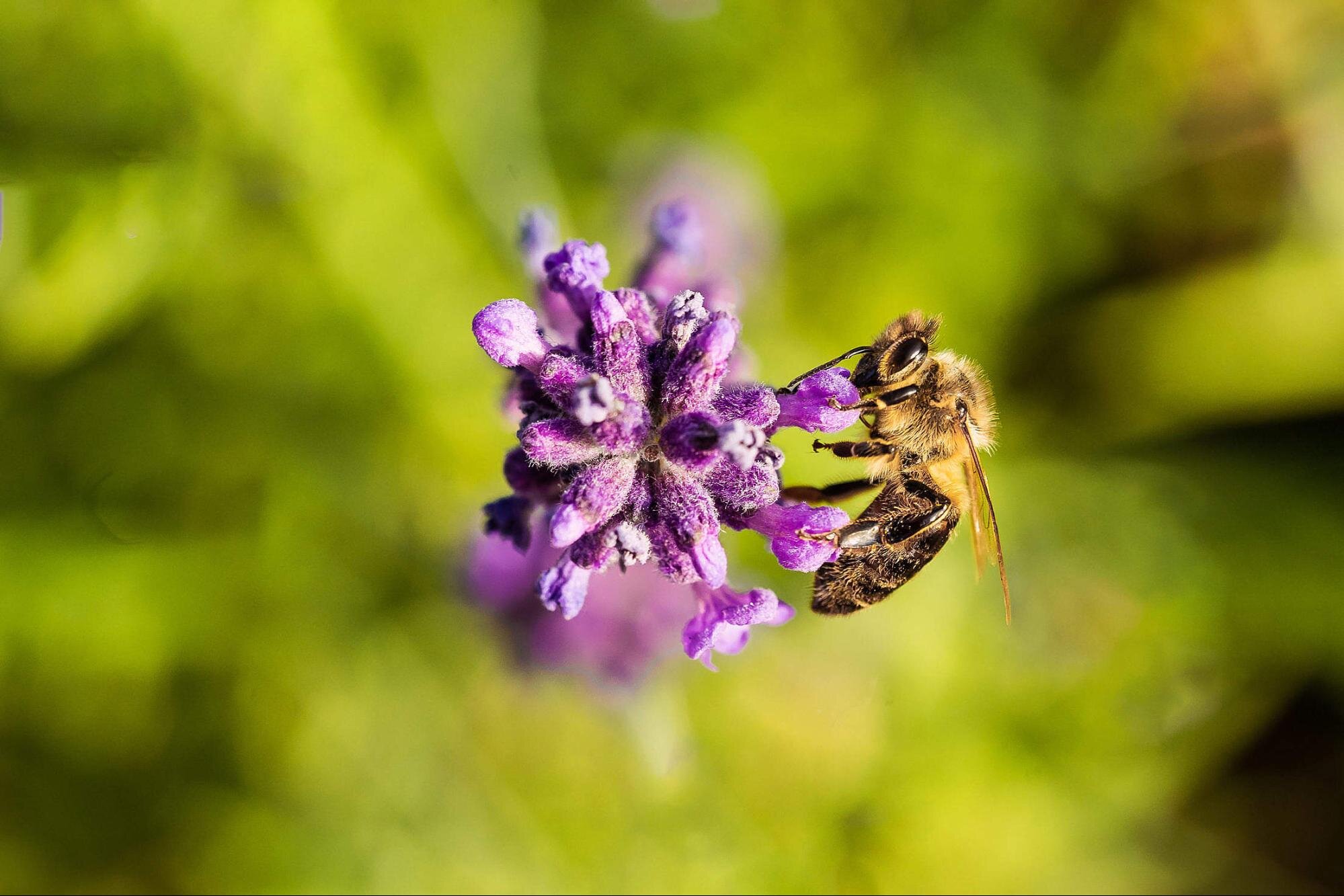The detailed photograph showcases a close-up view of a bumblebee resting on a complex purple flower, composed of numerous small blossoms or petals. The bee, featuring a black abdomen, a fuzzy white body, a dark brown head, and clear wings, is seen actively extracting nectar or pollen with its face immersed in the flower. Positioned on the right side of the flower cluster, the bee appears larger in size compared to the individual tiny flowers on which it feeds. The backdrop of the image is a blurred green expanse, presumably the leaves or lower parts of the plant, ensuring that the primary focus remains on the vibrant purple flower and bumblebee. The flower’s hue is a balanced shade of purple, neither too dark nor too light, and its intricate floral structure is reminiscent of plants like lavender, although it may not be one.